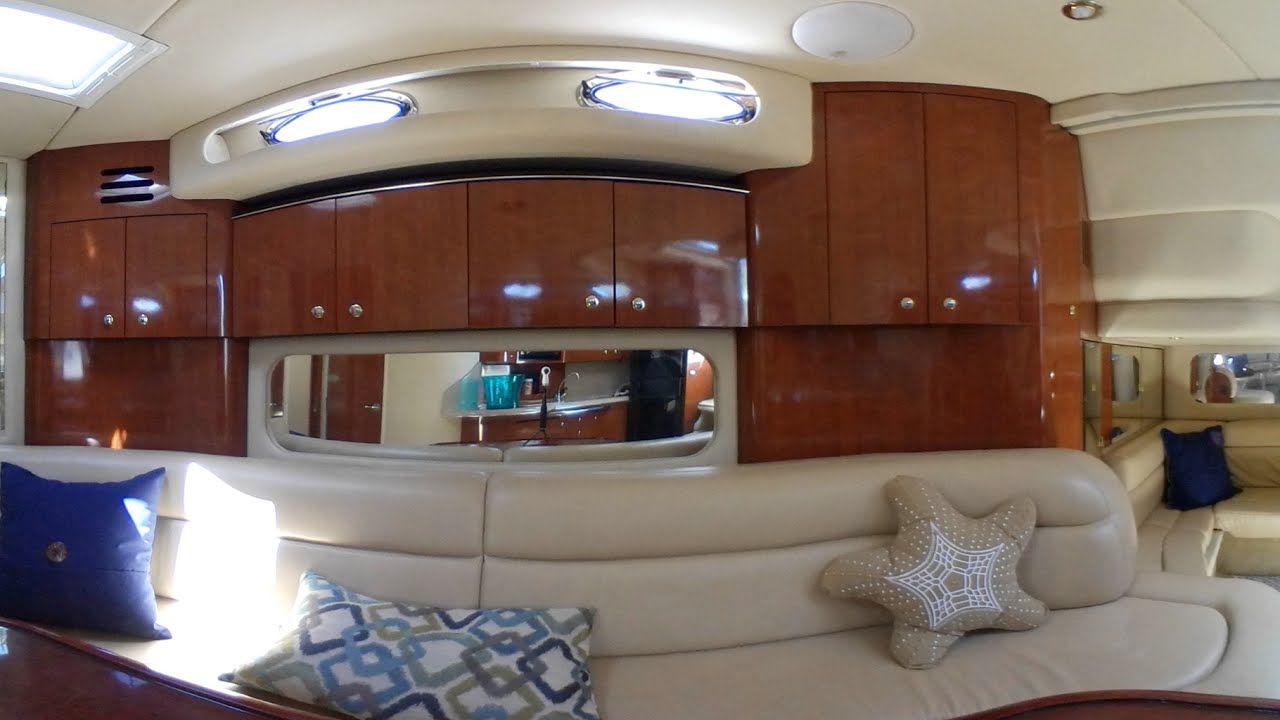The image showcases the luxurious interior of a likely high-end yacht. The space is adorned with shiny, light brown wooden cabinets that line the far wall, their reflective surfaces adding to the opulent ambiance. Centrally placed within the cabinetry is an oval-shaped mirror, which reflects the room's other side and further amplifies the feeling of spaciousness. Beneath the cabinets is a padded, white couch that stretches the length of the room, providing ample seating. The couch is decorated with nautical-themed cushions, including a prominent tan starfish-shaped pillow with a white spiderweb design and another blue pillow adorned with concentric rings. Above, the ceiling is painted white and includes both a round light and a rectangular window, contributing to the room's bright and airy feel. Completing the sophisticated look, there is a white outcropping with two round windows adding character and functionality. The room also features a kitchen area equipped with a fridge, cabinets, counters, and professionally arranged lights, underscoring the yacht's blend of luxury and practicality.